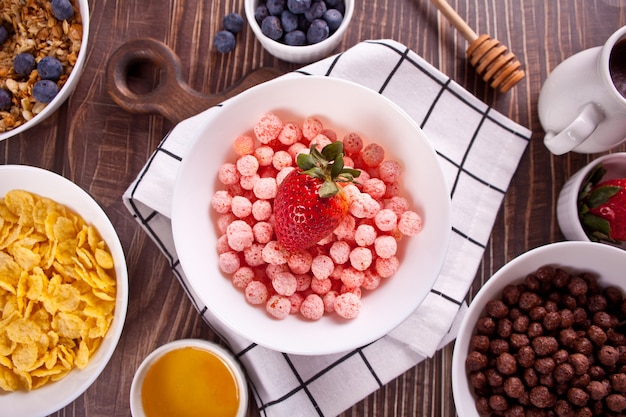The photograph captures an overhead view of a table covered with various types of cereal in different bowls. Centered on a black and white checkered tablecloth, which rests on a wooden trivet, is a white bowl of pink cereal balls with a strawberry perched on top. To its left, another white bowl appears filled with cornflakes. Between these two is a small condiment bowl containing honey. 

On the bottom right, there's a white bowl filled with Cocoa Crisp. Above it, a small bowl holds a single strawberry. Further up, in the top right corner, a white pitcher and a honey dipper suggest the presence of honey, indicated by the adjacent spiral honey spoon. Just above the central pink cereal bowl, a small condiment dish can be seen.

In the top left corner, a white bowl holds a dark brown cereal, possibly with blueberries. The scene is brightly lit, likely from natural lighting, enhancing the clarity and details of the various elements on the wooden surface, which could be either indoors or outdoors. There is no text within the image.